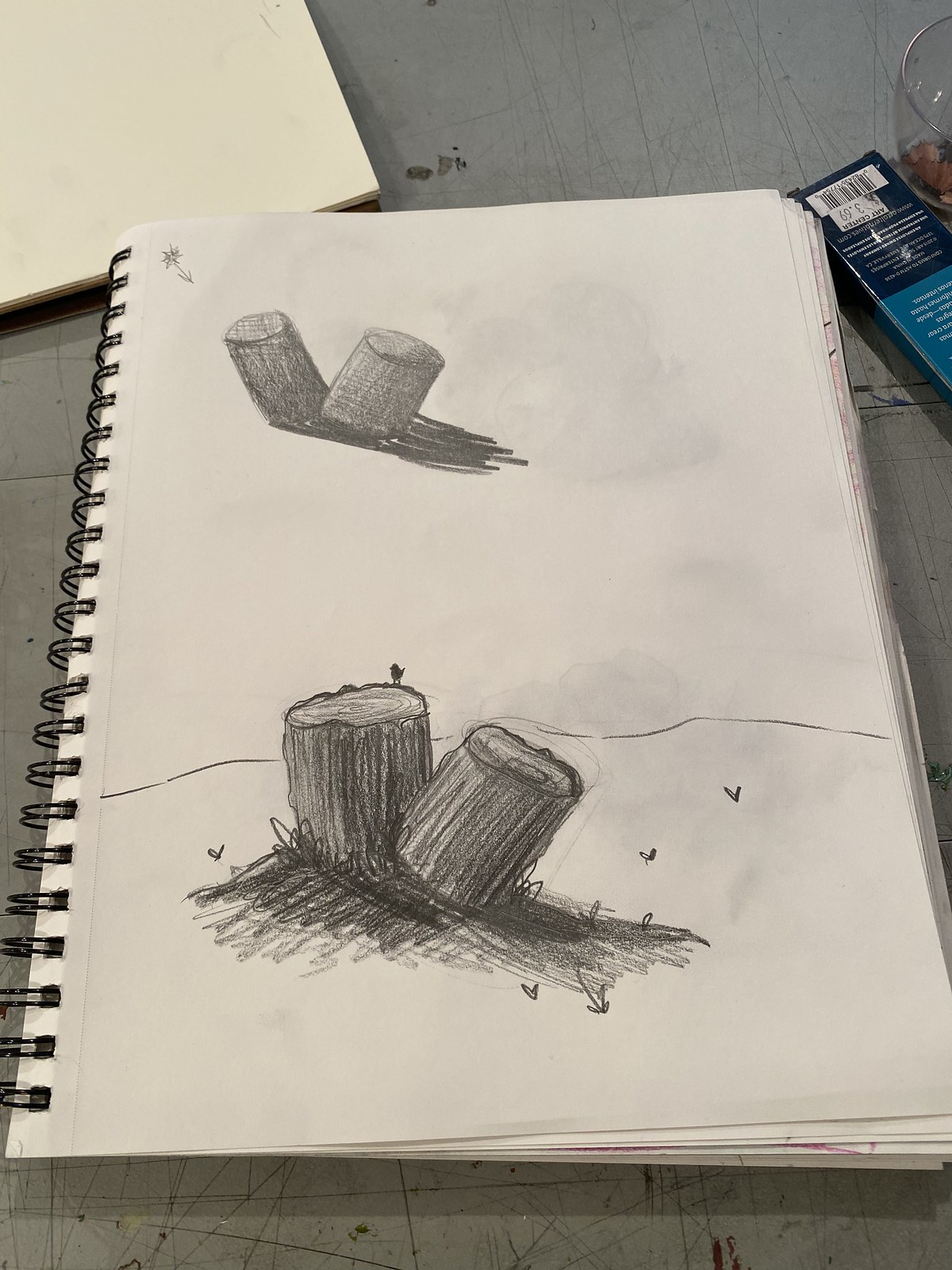A detailed photographic image depicts a sketchbook lying on a rough, gray table with visible scratches. The sketchbook, identifiable by its black spiral binding on the left, contains detailed pencil sketches. On the top portion of the page, there are two logs drawn diagonally with subtle shadowing and erase marks, giving them a lifelike texture. At the bottom of the page, another set of logs is illustrated, accompanied by additional shading and surrounded by motifs such as hearts, butterflies, and a bird flying above, giving a whimsical touch to the scene. To the upper left corner of the page, only a corner of another book or set of pages is visible, showing faint pencil markings. On the right side of the table, a blue box with white text and a price tag reading "Art Center, $3.69" along with a black and white barcode is also visible in the scene.